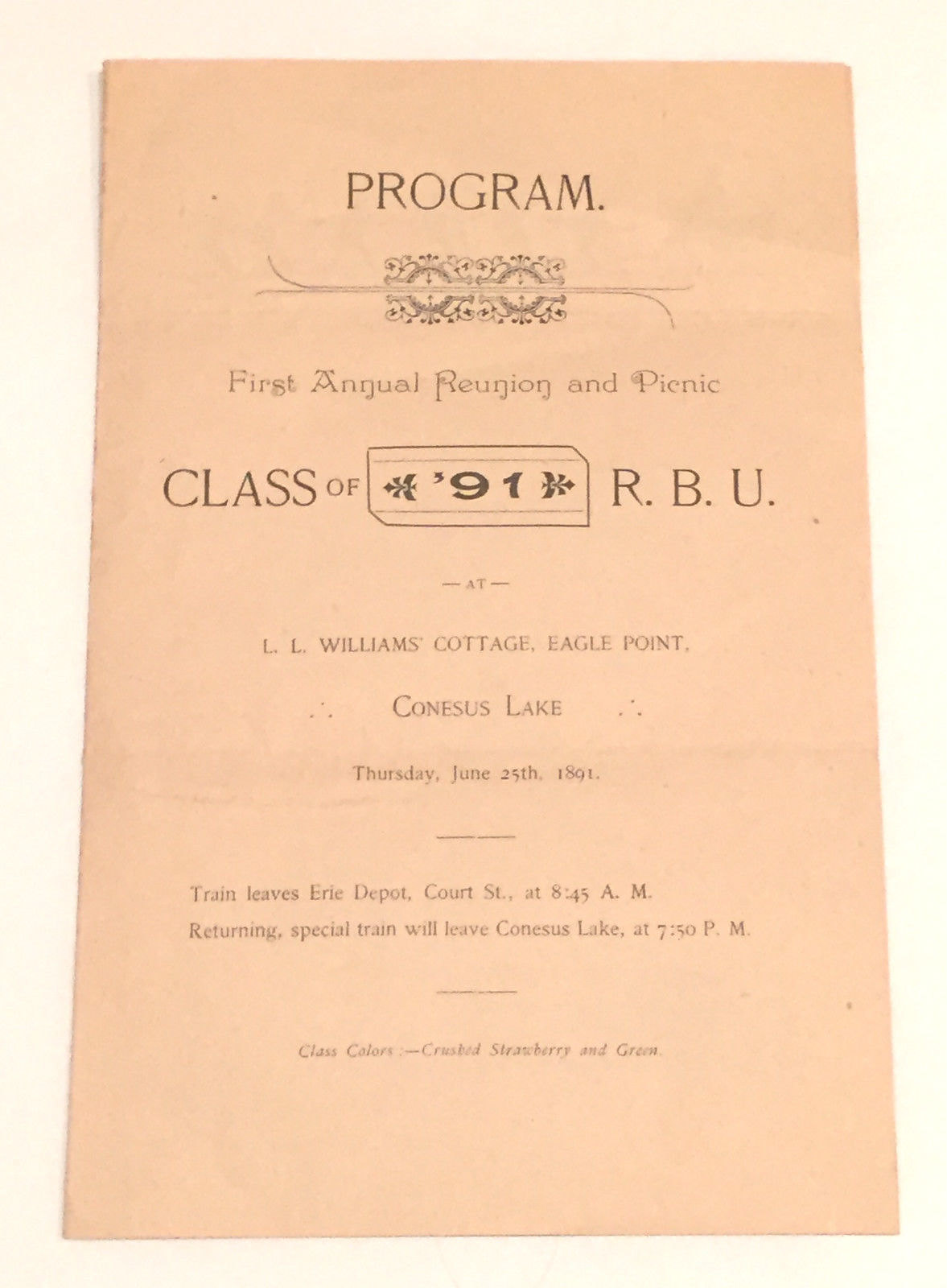This is a vertical rectangular program pamphlet from the first annual reunion and picnic of the Class of '91, RBU, an event held at L.L. Williams Cottage, Eagle Point, Constance Lake, on Thursday, June 25th, 1891. The program is a light sandy peach color against a very light yellow background, with black printing. At the very top, it reads "Program," followed by a decorative floral design. Below this, in fancy font, it states "First Annual Reunion and Picnic" and then in larger letters, "Class of '91, RBU." Further details include the location, time specifics—train leaves Erie Depot, Court Street, at 8:45 AM, with a returning special train departing Constance Lake at 7:50 PM—and the class colors, crushed strawberry, and green.